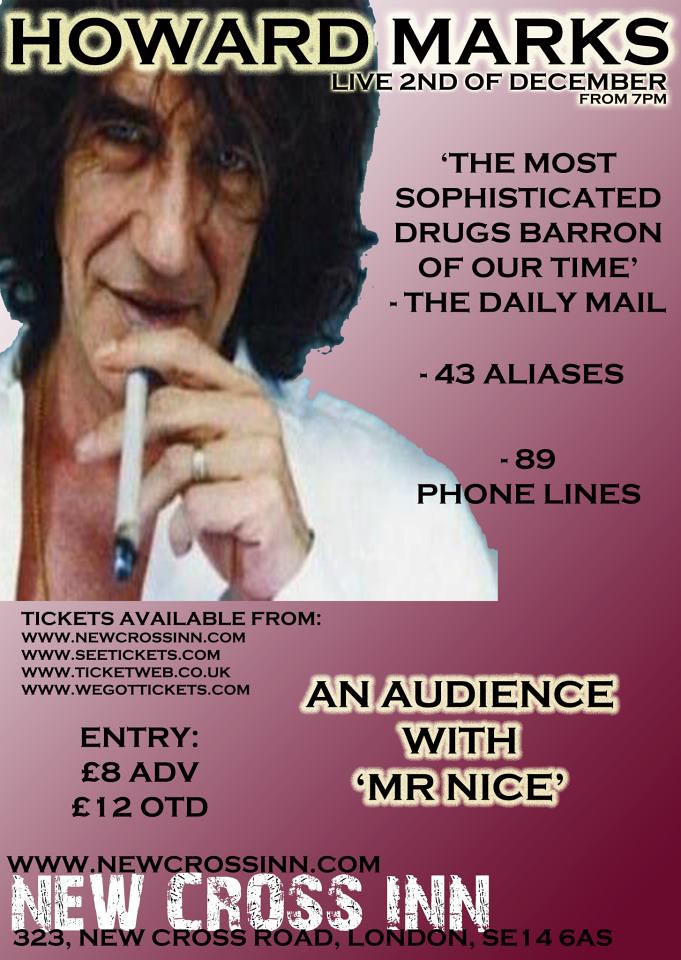The poster promotes a live show featuring Howard Marks on December 2nd at 7 pm. The background features a gradient pink color, transitioning from lighter pink in the top left to darker pink in the bottom right. Dominating the left side of the poster, there's an image of Howard Marks looking into the camera while smoking a cigarette, wearing a white long-sleeved shirt, a gold necklace, and a ring on his ring finger. Text to his right describes him as "the most sophisticated drugs baron of our time," referencing a quote from the Daily Mail, and notes his use of 43 aliases and 89 phone lines. The event is titled "An audience with Mr. Nice," and tickets can be purchased from various websites including newcrossin.com, ctickets.com, ticketweb.co.uk, and wegottickets.com. Entry is £8 in advance and £12 on the door. The venue is listed as 323 New Cross Road, London, SE14 6AS.